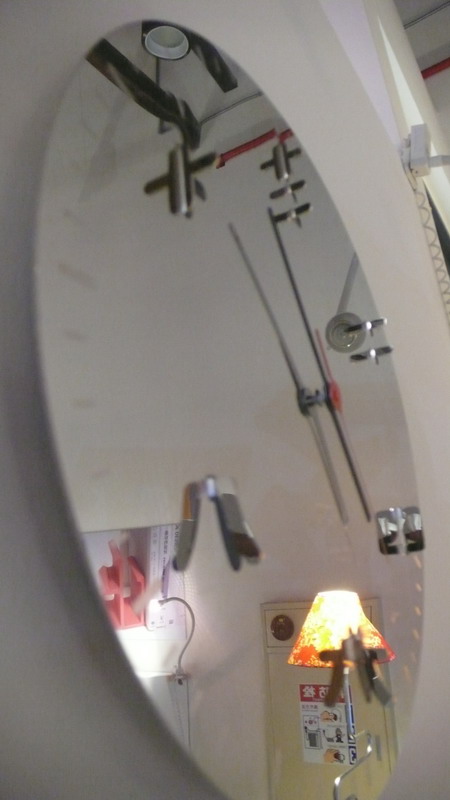This photograph captures a large round mirror mounted on a white wall, viewed from a side angle. The mirror's reflective surface reveals various objects. Dominantly, there are clock hands at its center, pointing as though part of a timepiece integrated into the mirror's design. The reflection shows diverse elements of the room: a silver-based lamp with a lit lampshade in the bottom right, a photograph or painting depicting a pink flower slightly above and towards the left, and a light fixture with a black exterior and white interior hanging from the ceiling. Additional items include a calendar, what appears to be a poster with illustrated rescue techniques, and various metal tubes and objects scattered throughout the room. The image also captures some red trim and a whiteboard in the top right corner, along with a mounted white box. The intricate details painted through the mirror's reflections suggest a complex, multifaceted room, potentially a bathroom, filled with eclectic items and a visually engaging arrangement.